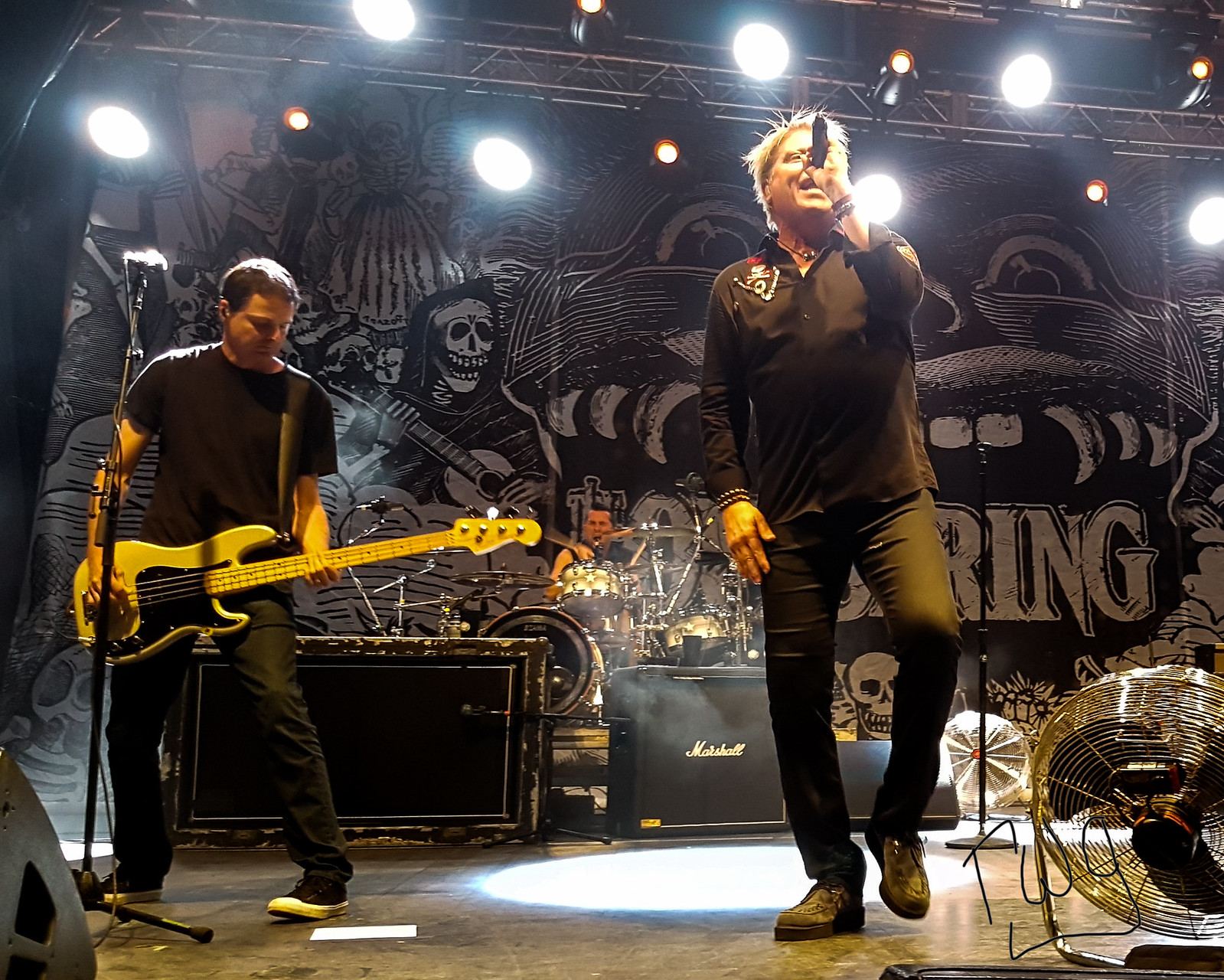The image captures a dynamic performance of a musical band on stage. The setting is a dimly lit stage with various spotlights shining from above, creating an intense atmosphere. The backdrop features a striking black and white illustration, depicting a skeletal figure in a black hood—resembling the Grim Reaper—holding a guitar. Surrounding this central figure are additional skeletons and a menacing creature with an open mouth, fangs, and bulging eyes. Partial lettering to the right spells out "R-I-N-G," while the rest is obscured.

In the foreground, the lead singer stands to the right, mid-performance, gripping a microphone with his mouth open, immersed in his vocals. He has spiky blonde hair and is dressed in a black, long-sleeve button-up shirt and dark pants. To the left, the bassist is playing an electric bass guitar, clad in a black short-sleeve shirt and dark pants. Both musicians are positioned in front of fans encased in chrome cages, although these appear to be inactive. Behind them, barely visible among the speakers and stage equipment, a drummer can be seen playing a drum set. The stage setup includes metal bars and possibly a catwalk overhead, enhancing the industrial vibe of the scene.